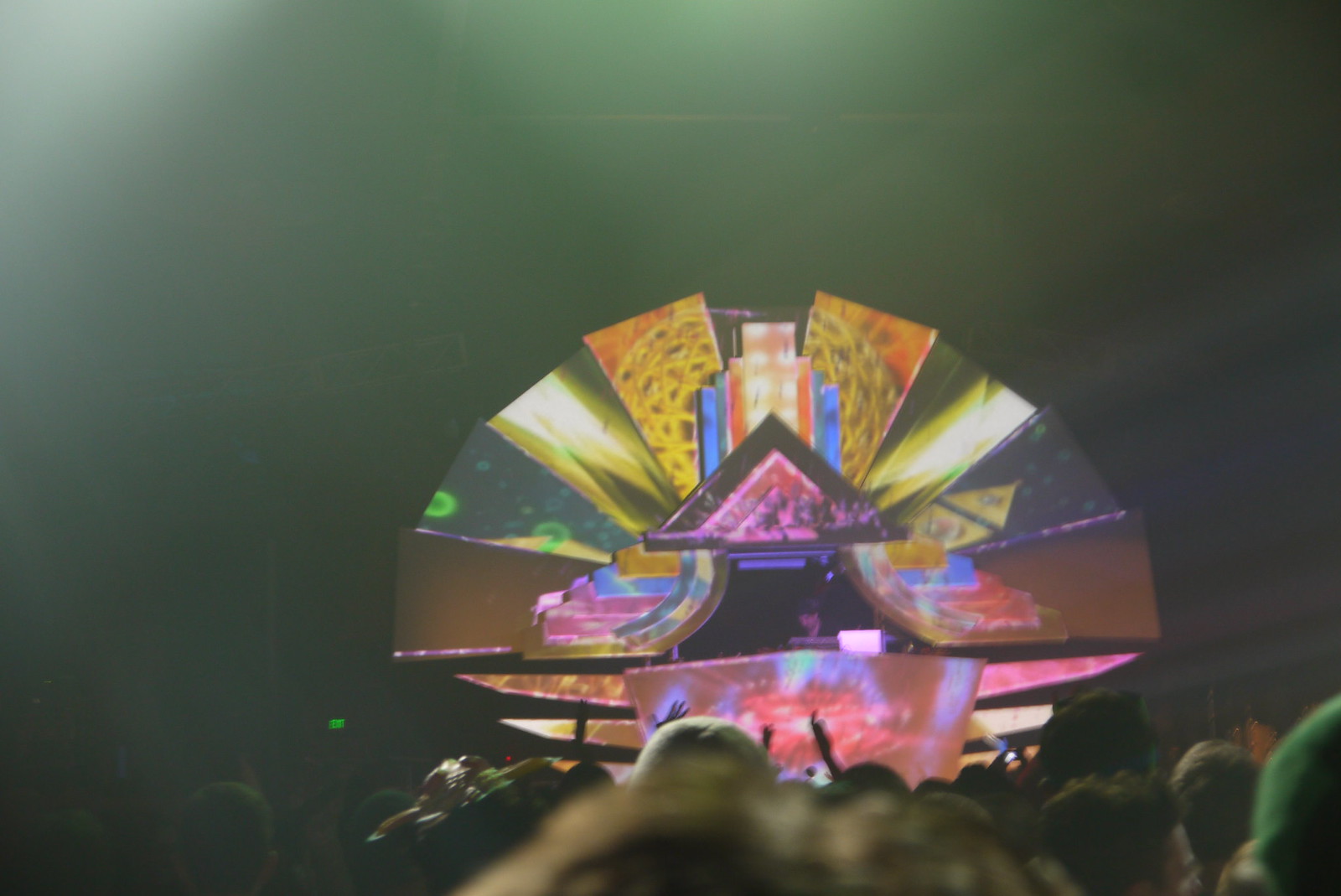This image features a vibrant, colorful scene from an electronic music concert or rave. The photograph captures the view of a crowd with their hands up, cheering and watching the stage. The stage is adorned with a striking, abstract, and geometric art installation, characterized by vivid hues of pink, yellow, green, and orange. The central figure on stage is a DJ, immersed within this intricate, science fiction-like set piece composed of various shapes, including triangles and rectangles. The background is muddled, with a greenish hue contributing to the overall chaotic and lively atmosphere, enhanced further by hazy, fog-like lights. The ensemble creates an exciting, almost surreal visual experience that blends music and modern art.